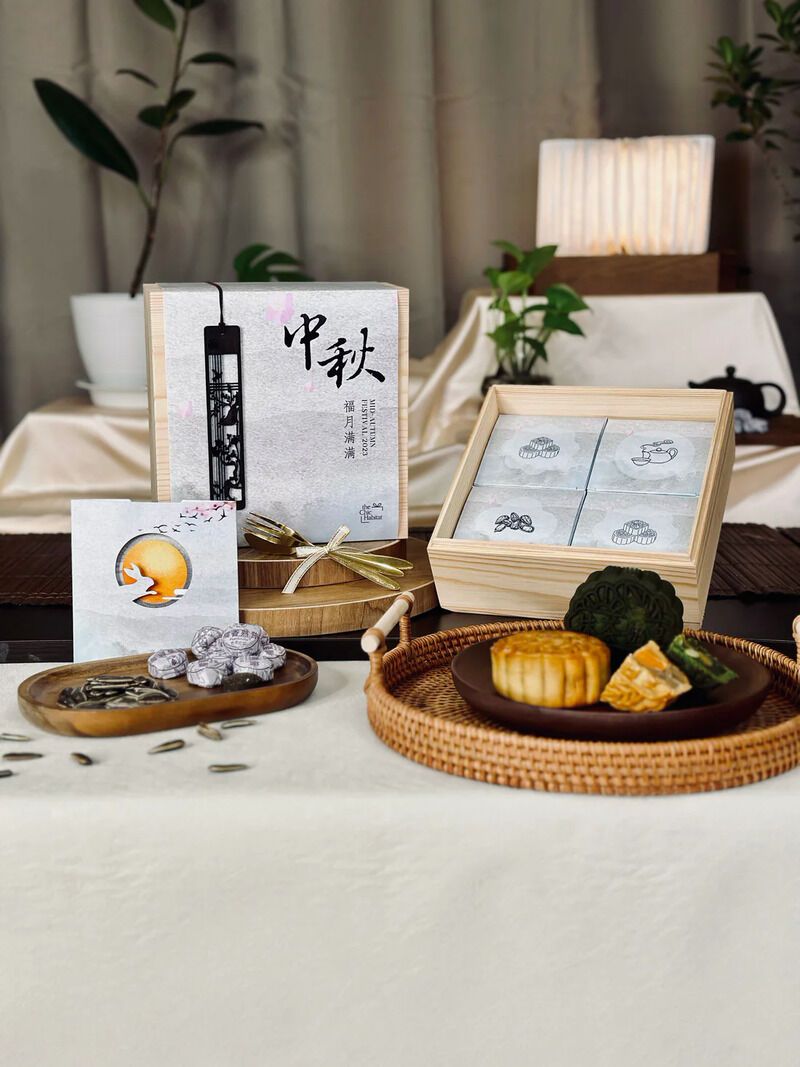The image showcases a luxurious and regal arrangement of assorted East Asian treats, prominently featuring a selection of moon cakes typically exchanged during the Lunar Festival. Displayed are two boxes of moon cakes, each offering an assortment of flavors, with visible varieties including a dark green flavor and a traditional baked version, meticulously placed on a brown plate within a basket-style serving tray. The setting oozes sophistication, with an off-white, silky draped background, complemented by lush green houseplants and a sleek black teapot that adds a touch of elegance. The main focus is on a refined light brown wooden box adorned with Japanese characters, containing four small paper packages, suggestive of a Japanese brand presenting an array of sweets and small seeds delicately encased within. The arrangement rests on a white tablecloth, positioned in a setting that is carefully styled to exude upscale aesthetics, highlighted by a grey curtain and a soft, bright studio-like lighting that slightly illuminates a small paper lamp in the background. Additional elements include a small wooden board with a coffee setup at the bottom right of the wooden box, contributing to the refined and curated ambiance of the display.